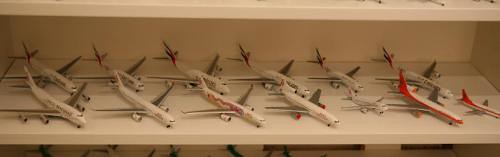In this color photograph, 13 miniature airplane models are meticulously arranged on a long, white shelf. The front row features seven planes, while the back row is composed of six. All the models boast gray wings and predominantly white bodies, with varying degrees of red accents. Notably, two airplanes on the right corner, as well as two in the center-front, showcase more prominent red stripes along their sides. The collection includes two smaller planes in the front row: one in the far right corner and another third from the right. These two differ from the others, which resemble large commercial jets. The shelf appears to have multiple levels, though only the top ledge and a glimpse of the lower row are visible, hinting at an extensive and detailed collection.